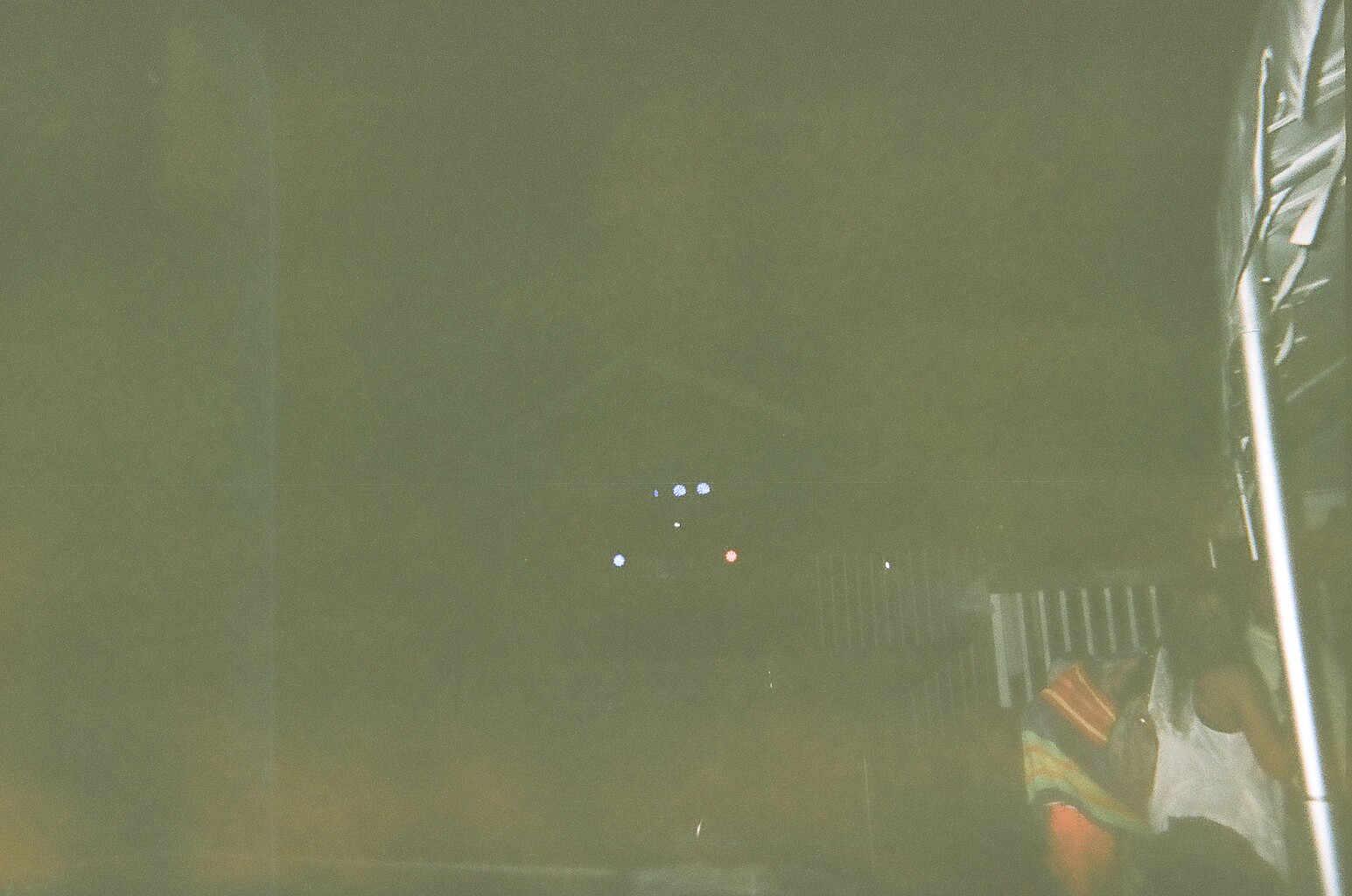In this nighttime photograph, the environment is cloaked in darkness, creating a scene with an overall greenish haze—the result of the camera's adjustment to low light conditions. Towards the bottom of the image, an orange haze gradually transitions into the dominant green hue higher up. In the distant background, a structure with a white-colored triangular arch, likely the roof of a building, is faintly visible.

Prominent in the scene are three blue lights accompanied by another set of blue and red lights, likely belonging to a large vehicle such as a semi-truck, fire truck, or ambulance, positioned across the way. Some guard rails or fencing can also be discerned in the further distance.

In the middle ground, a woman dressed in a white top stands beside a multicolored towel that features red, yellow, blue, and green segments, adding vibrant splashes of color to the otherwise dim setting.